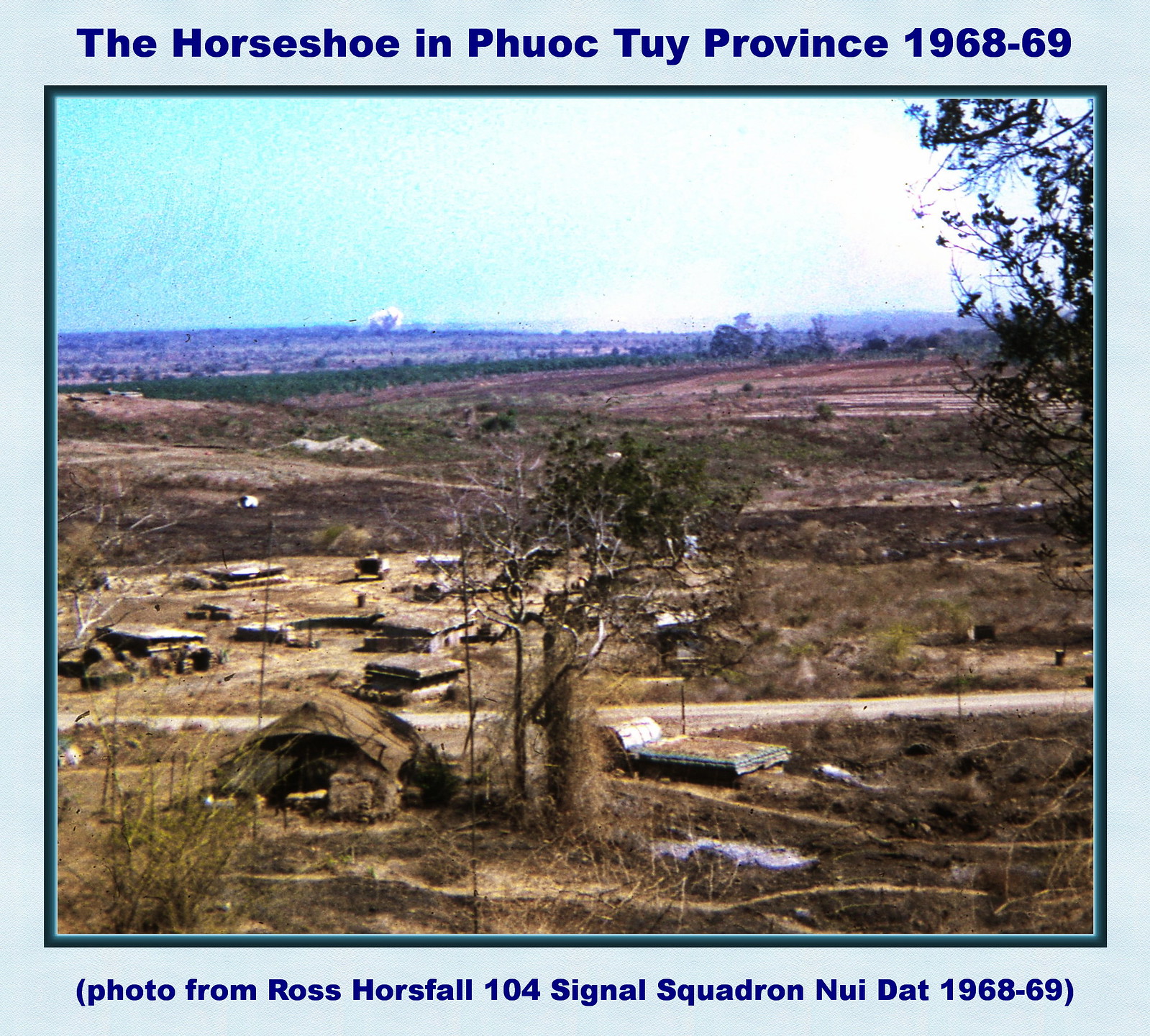The square-shaped image, bordered with a light teal trim, depicts a rural landscape titled "The Horseshoe in Phuoc Tuy Province, 1968-69" in dark blue letters at the top. Below this title, the text in parentheses reads, "Photo from Ross Horsefall, 104 Signal Squadron, Nui Dat, 1968-69." The image shows a mostly barren terrain, with patches of dirt and sparse grass covering the flat expanse. The foreground features a few brownish huts and makeshift structures, along with some debris that might be trash or part of a tent. A thin dirt road stretches horizontally across the lower part of the photo. Additional details include scattered shrubby trees on the right, a small tree in the center, and some tall buildings faintly visible in the distant background. The sky covers the upper third of the photo, transitioning from a grayish haze on the right to a light turquoise blue on the left, giving a sense of depth and atmosphere to the scene.